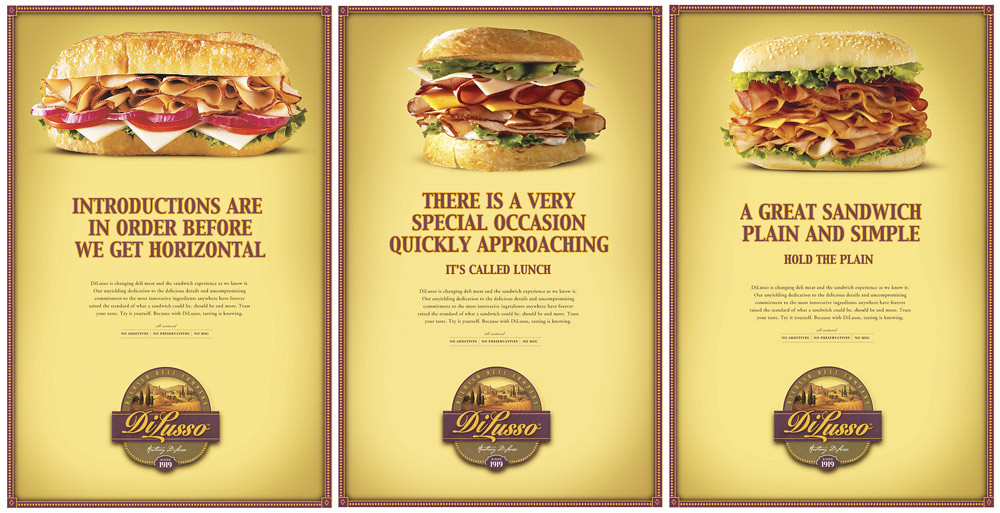The image is a three-panel advertisement for Di Lusso, each panel featuring a different sandwich against a yellowish tan background with distinctive red borders adorned with white dots. At the top of each panel, there's a sandwich: the left panel showcases a turkey sub, the center panel displays a circular roast sandwich, and the right panel features a sandwich with a lighter sesame seed bun, possibly with bacon, ham, or turkey. Each sandwich section contains bold text in brown print. The left panel reads, "Introduction are in order before we get horizontal," while below is an illegible paragraph. The center panel states, "There is a very special occasion quickly approaching. It's called lunch." The right panel says, "A great sandwich, plain and simple, hold the plane." At the bottom of each panel is the Di Lusso logo, which includes a rounded arch with an image of a country hillside inside it, outlined in plum color. Below that is a purple banner with "DeLusso" in yellow print, and another blurry text written in white over a gray background. Finally, at the very bottom, there is a purple circular stamp that reads "1919." The vibrant colors, clear spacing, and detailed design elements strongly suggest it's an advertisement for a sandwich shop.